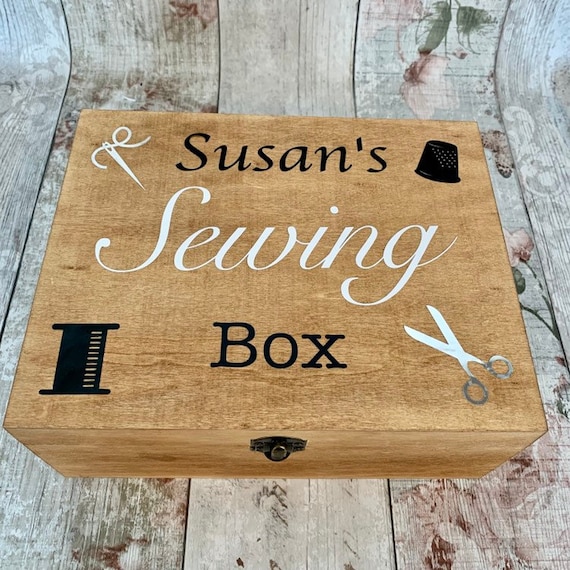This up-close home decor photograph features a medium-colored wooden box labeled "Susan's sewing box." The text on the box is distinct: "Susan's" at the top in black, "sewing" in white cursive in the center, and "box" in black at the bottom. The top of the box is adorned with various sewing-related illustrations: a sewing needle with thread in the upper left corner, a thimble in the upper right, a pair of scissors in the bottom right, and a spool of thread in the bottom left. A small hook latch is visible at the bottom of the box, though it lacks an actual lock. The box is placed on a very light grayish wooden surface, almost white, which might be a bench or table, adorned with painted pink blossoms and green leaves. The overall ambiance of the scene suggests a charming and nostalgic workspace for sewing.